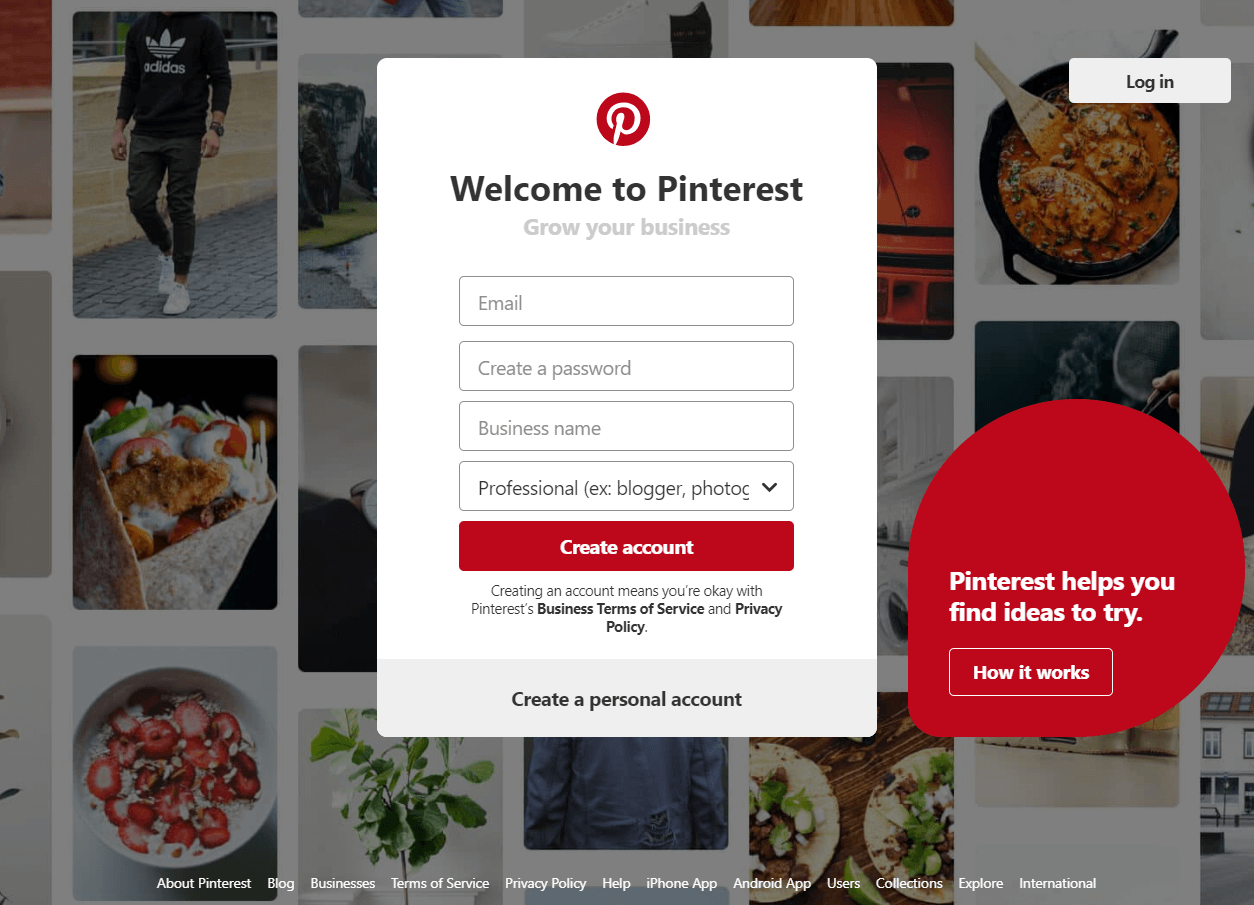Screenshot of a Pinterest Sign-Up Page:

The image captures a sign-up page on Pinterest's website. The page features a pop-up sign-up form centered against a subtly darkened collage background. The backdrop includes an array of images such as food items, clothing articles, landscapes, and vehicles, all uniformly softened with rounded corners and laid over a white base.

Dominating the center, the white pop-up form is accentuated by a gray footer. At the top of the pop-up is a dark red circle encasing a white "P", the Pinterest logo. Below this emblem is the welcoming phrase "Welcome to Pinterest" in bold black lettering, followed by the phrase "Grow your business" in small gray text.

The form progresses with four text entry fields, each outlined with a thin gray line and placeholder text. The fields read as follows:
1. Email
2. Create a password
3. Business name
4. Professional (e.g., blogger, photographer), partially cut off, with a gray downward arrow button indicating a dropdown menu.

Beneath these fields is a prominent, slightly rounded red button labeled "Create account" in white text. Further down, in smaller gray print, is a disclaimer: "Creating an account means you're okay with Pinterest's Business Terms of Service and Privacy Policy," with the latter phrases in bold for emphasis.

To the right side of the sign-up form, a bright red, uniquely shaped element with a rounded corner on its bottom left displays the message "Pinterest helps you find ideas to try" in white text. Below this message is a white button that reads "How it works."

The overall emphasis of the screenshot highlights the user-friendly and visually cohesive design of Pinterest's sign-up page, encouraging new users to create a business account.